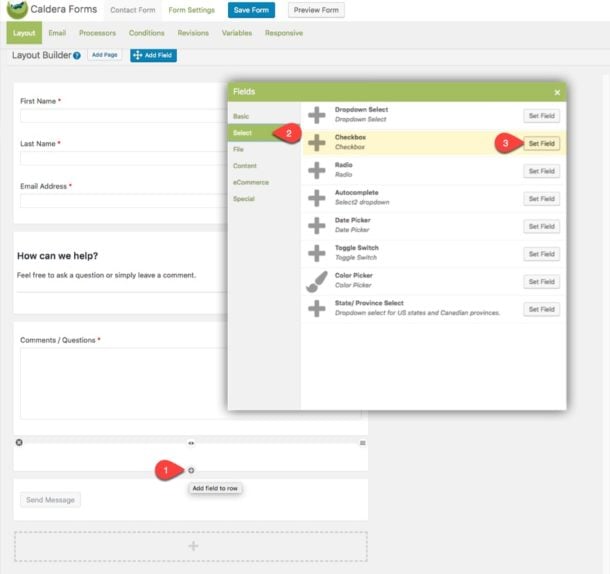The image is a detailed screenshot of a website page titled "Caldera Forms." In the upper left corner, the Caldera Forms logo is prominently displayed. Below the header is a navigation bar featuring several menu items including "Contact Form," "Form Settings," and a blue "Save Form" button alongside a gray "Preview Form" button.

Further down, a secondary navigation bar is present, starting with the "Layout" tab highlighted in green. Options such as "Email," "Processes," "Conditions," "Revisions," "Variables," and "Responsive" are also listed. 

The main section of the screenshot is the "Layout Builder" interface, featuring controls for adding pages and fields. Visible within the builder is a form outline consisting of input fields labeled "First Name," "Last Name," and "Email Address." Below these fields is a text prompt stating, "How can we help? Feel free to ask a question or simply leave a comment," followed by a large rectangular comment/questions box.

Towards the bottom, a slider control is visible, with options to "Add Field to Row" and a "Send Message" button that is grayed out. On the right, an open menu labeled "Fields" in green contains various input options such as dropdown select, checkbox, radio button, auto-complete, date picker, and toggle switch. Next to the checkbox option, there is a "Set Field" box marked with a small red dot containing the number "3."